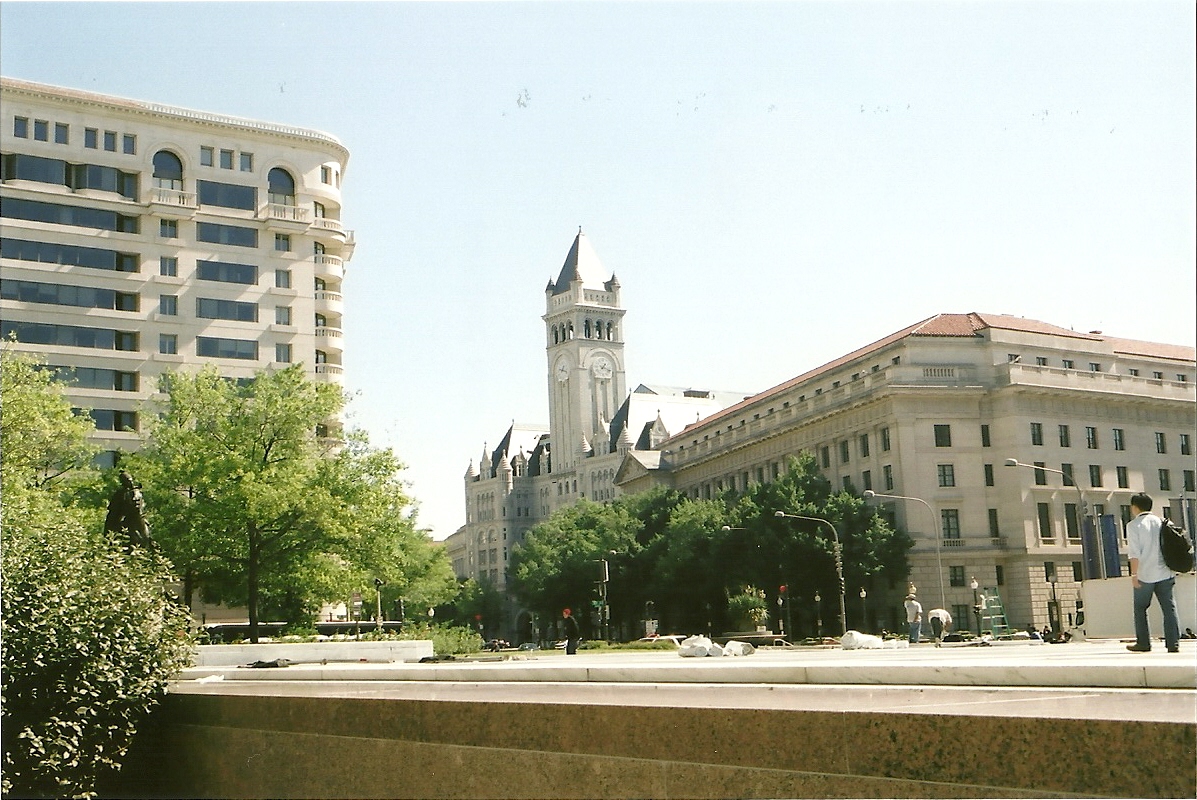In this city scene captured on a clear, cloudless day with a vibrant blue sky, a bustling street divides two distinct architectural landmarks. The foreground is anchored by a white, polished marble sidewalk running alongside a two-lane road, which is bordered by a stone wall. On the right side of the image stands a grand old building with cream-colored stone walls and a distinct clock tower capped with a pointed, reddish-orange roof. This building exudes a historic, almost castle-like charm. 

Towards the left, across the street, a taller, modern skyscraper rises, featuring sleek glass windows and a minimalist white facade. In front of this building, a park-like area filled with greenery and shrubbery partially obscures a bronze statue or public monument. Amidst the urban backdrop, a few pedestrians are scattered along the walkway: a young man in his mid-twenties with a backpack, white shirt, and jeans walks away from the camera; nearby, another person, who appears to be male, stands wearing jeans and a hat while a third person bends over, their details indistinct. Trees with lush green leaves are interspersed around the scene, casting their shadows. Traffic lights and streetlights punctuate the road, adding a touch of modernity to this otherwise historic and serene urban landscape.